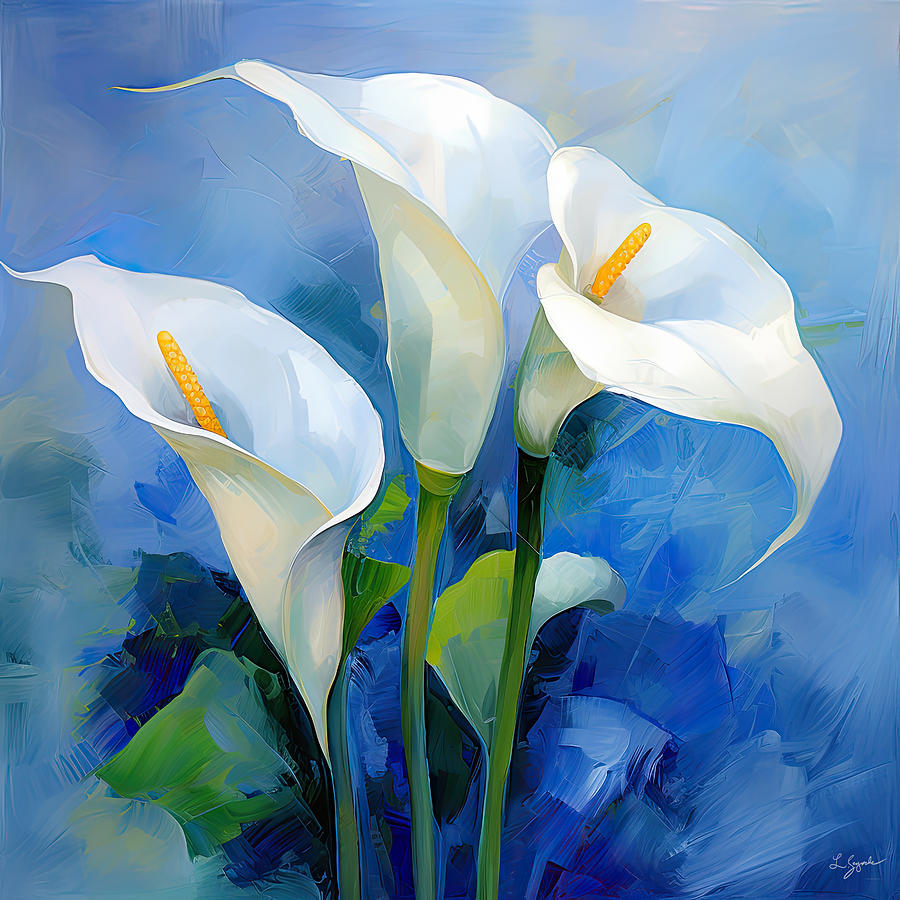This is a vibrant acrylic painting depicting three white peace lilies with cupped blossoms and yellow-gold pistils at their centers. The flowers stand prominently in the middle of the canvas, each supported by lush, green stems and accompanied by a few green leaves. The background features a dynamic blend of blue hues, transitioning from deeper blue shades at the bottom to lighter blue at the top, applied with broad brush strokes that convey a sense of movement and depth. The painting's texture enhances the lifelike quality of the lilies, making them appear healthy and hydrated. An artist's cursive signature is delicately placed in the lower right-hand corner. This impressionistic work beautifully captures the elegance and vitality of the peace lilies.